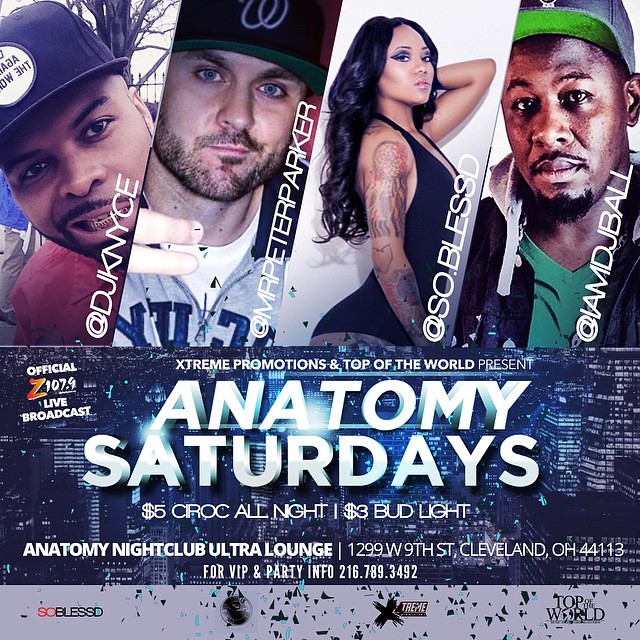This promotional flyer for an upcoming music event is visually engaging and features a split design with rich details. The upper half of the flyer is devoted to four diagonal-framed photographs of the event's performers. The first image, from left to right, is of a young African-American man wearing a black baseball cap with a white circle logo, showing a gold grill in his teeth and a red shirt. His name, "@DJANYCE," is displayed in vertical white text over his image. Next is a young Caucasian man in a gray zip-up hoodie over a white t-shirt, and a black cap with a white "W." His name, "@MRPETERPARKER," appears in similar vertical white text. To his right, there is a dark-haired young woman with long hair parted in the middle, posing in profile while wearing a tight black evening dress with thin stripes. Her heavily tattooed right arm is visible, and her name, "@SOBLESSD," is indicated in white vertical text. The final image showcases an older black man in his thirties wearing a green-billed baseball cap, a black and white jacket with a hood, and a green t-shirt. His name, "@IAMDJBALL," is presented in vertical text.

The lower half of the flyer features a dark blue background depicting an aerial view of a cityscape. At the top of this section, bold white text reads "Extreme Promotions and Top of the World Presents." Beneath, larger 3D white text announces "Anatomy," italicized, while parallel text reading "Saturdays" is non-italicized. The subsequent lines highlight special offers with "$5 CIROC all night" and "$3 Bud Light." Further details include "Anatomy Nightclub Ultra Lounge," along with the address "1299 West 9th Street, Cleveland, Ohio, 44113," and a line for VIP and party information at "216-789-3492." The lower left corner has the logo "Official Z-107," indicating a live broadcast, while the bottom section, splattered in gray ink, includes the names "So Bless," "Extreme," and "Top of the World." The flyer is segmented by small blocks and bars that enhance its organized look.